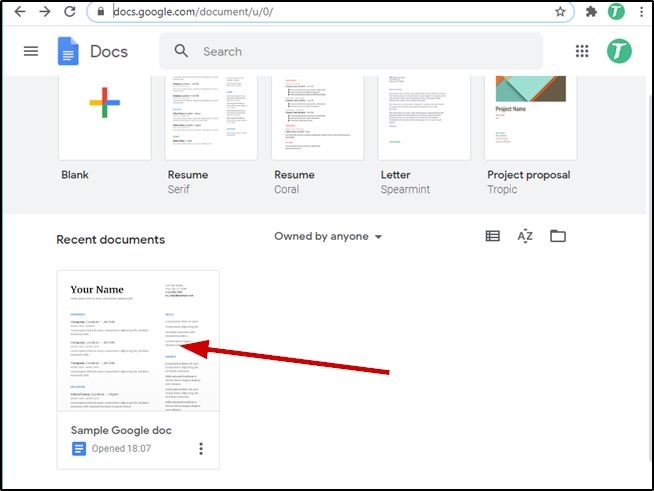The image depicts an open Google Docs website with a white background, displayed on the URL 'docs.google.com'. At the top left is the Google Docs logo featuring a blue document icon followed by the word "Docs". The interface includes a multi-colored 'Blank Document' icon, comprising a red plus sign on top, yellow on the left side, blue on the right side, and green on the bottom.

On the screen, five templates are visible. The first template reads 'Blank' and is indicated by the plus sign icon. The second template is titled 'Resume (Serif)' and includes a thumbnail image of a resume. The third template, 'Resume (Coral)', is placed immediately to the right of the second. The fourth template is 'Letter (Spearmint)', and the fifth is titled 'Project Proposal'.

Below these templates are tabs like 'Recent Documents' and 'Owned by me'. A document named 'Your Name' is displayed as a sample of a resume or template. An arrow, colored red, points from the center of the screen to the bottom left, highlighting this document. The time notation '18:07' appears to indicate when the document was last accessed or created.